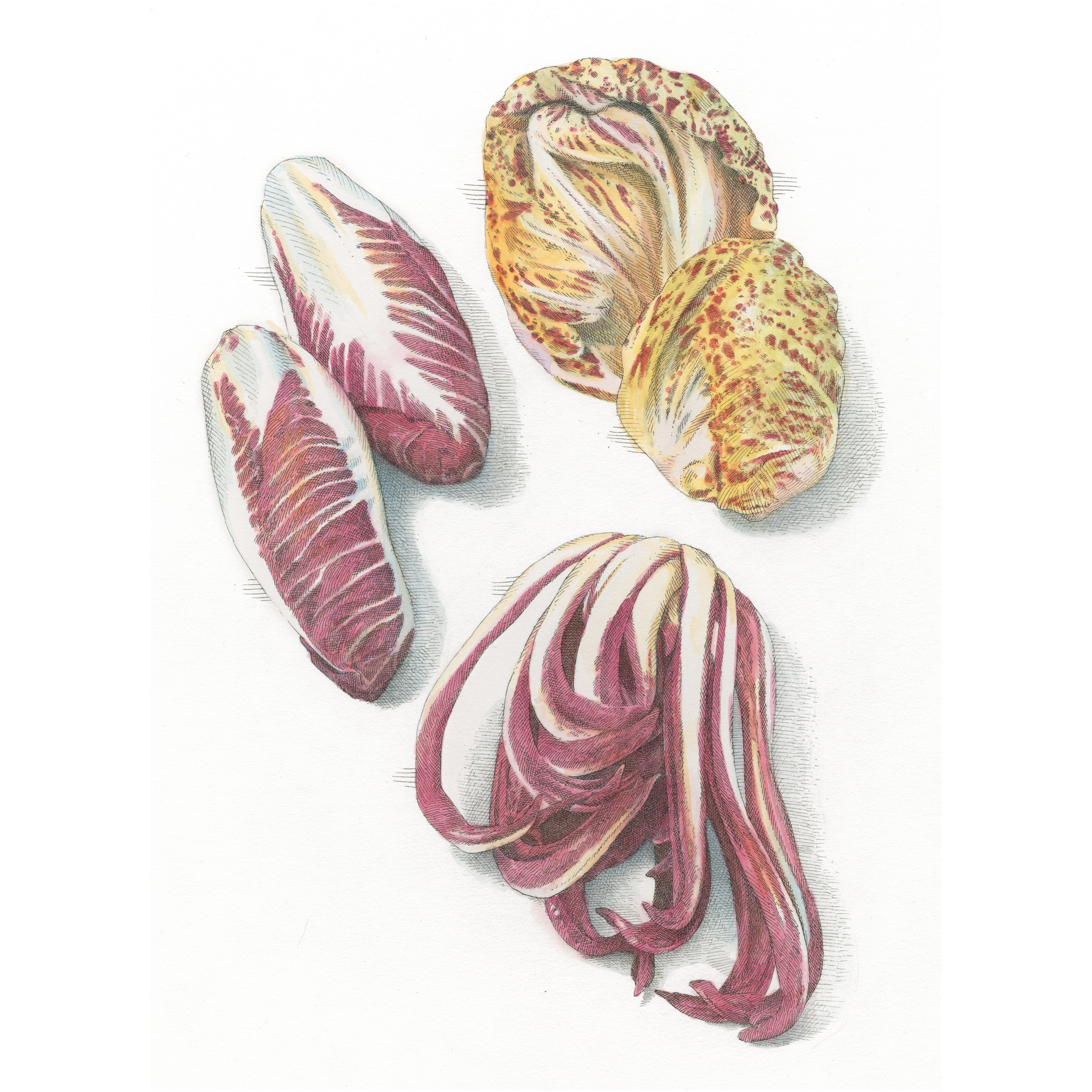This image is a soft yet realistic illustration featuring various organic forms that resemble both flower petals and anatomical structures. The background is white, making the muted and intricate colors stand out. In the upper left section, two oblong shapes, extending with veins like cabbage, display a transition from white to reddish-purple hues. To the upper right, a circular figure smushed in appearance exhibits speckles of yellow, burgundy, and white. Below it, a rounded shape with the same colors evokes the texture of a head of lettuce. Finally, on the bottom, there are tentacle-like forms with strips of white and burgundy, contributing to the diverse shapes and textures seen throughout the image. These elements blend to create a striking composition that bridges the natural beauty of flower petals with the complexity of organic anatomy.